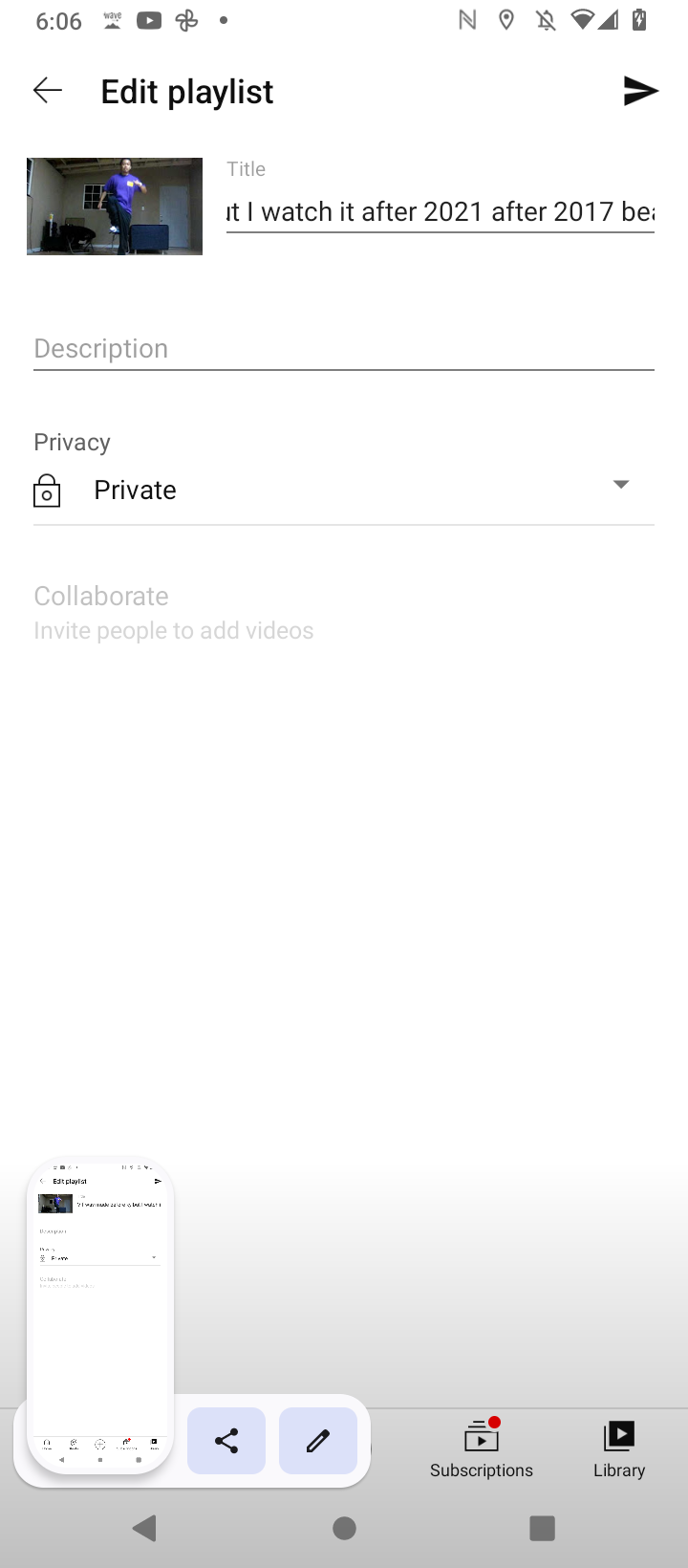This image is a tall, narrow screenshot that appears to be taken from a mobile device, showing the interface of a playlist editing feature, likely from a music or video streaming app. The layout is in portrait orientation, reflecting the dimensions of a phone screen.

At the top left corner, the text "Edit Playlist" is prominently displayed in black letters. Just below this, there is a small, somewhat indistinct image of a person wearing a blue shirt, seemingly jogging or running in a dimly lit environment.

To the right of this small image, the word "Title" is written in gray letters, with a list of partially visible text entries underneath, including "it," "I," "watch it," "after 2021," "after 2017," and "be." The rest of the text trails off and is not fully visible in the image.

Beneath this section is a gray line, followed by the word "Description" in gray text. Adjacent to this is the word "Privacy," along with an icon resembling a padlock, indicating that the playlist is set to private.

Further down, the word "Collaborate" appears in faint gray text, alongside the instruction "invite people to add videos," implying a feature for collaborative playlist creation. Below this is a large, blank white space.

At the very bottom, there's a gray footer area. This section includes a miniature version of the upper layout, with a long white bar and gray squares containing two icons: one with three dots connected by lines forming a 'V', and another resembling a marker.

To the right of these icons is a black button labeled "Subscriptions," followed by a play button with a small red dot above it. Adjacent to this is another black play button with the word "Library" beneath it. Completing this section are additional icons, including a stop play button and a circular button, possibly meant to signify an exit or logout function.